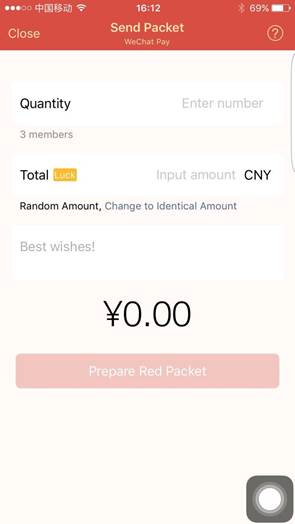The image appears to be a detailed screenshot of a mobile phone display, likely from a messaging or payment app. The top part of the screen features a prominent red rectangle, probably serving as a header or notification bar. In the upper-left corner, there is an icon representing "clothes" in white, followed by the time displayed as "16:12" (or 4:12 PM). Below this, another white icon labeled "Send Packet" is visible, which likely pertains to the WeChat Pay service. The phone’s battery icon indicates a 69% charge in white.

Further down, there is a circular outline with a red background and a white question mark in the center. The background color of the screen transitions to a lighter shade of red, creating a soft gradient effect. A white rectangle stretches across the screen, containing multiple text elements. On the left side of this rectangle, "Quantity" is written in black, with another text box in gray labeled "Enter Number" using capitalized initials.

Below "Quantity," it states "3 members," followed by some spacing and another white rectangle. This rectangle has "Total" written in black and is adjacent to an orange rectangle labeled "Luck." The following gray text box prompts "Input Amount," with "CNY" (Chinese Yuan) written in black capital letters next to it.

Underneath, the left side bears the text "Random Amount, Change to Identical Amount" in black. Further, there is another white rectangle containing the phrase "Best Wishes!" in gray, and below this, a numeric display reads "0.00" in black.

At the bottom of the screen, there is a red rectangle with white text that reads "Prepare Red Packet." The entire interface seems designed for initiating a payment or sending money, complete with options for specifying amounts and offering well-wishes.